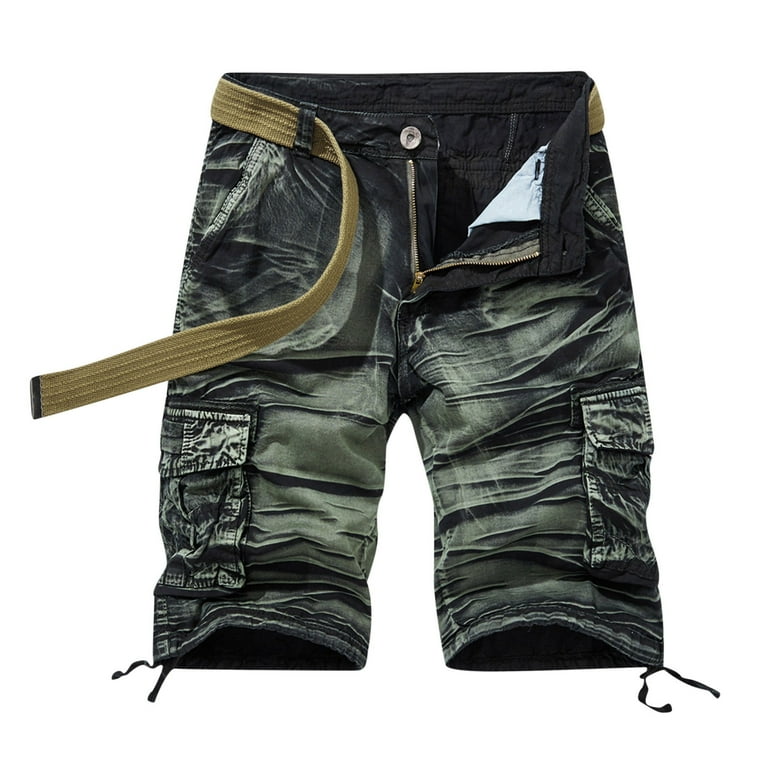This is a close-up photograph of a pair of weathered cargo Bermuda shorts. The shorts have a distressed, denim-like appearance with a variegated color ranging from navy to a greenish-bluish-gray, giving them a unique, worn look. The fabric appears wrinkly and weathered, with washed-out white splotches that accentuate the original jean material, particularly noticeable on the large, flap-closure pockets on the outer thighs. Each pant leg features additional pockets toward the end, with these pockets occupying almost a third of the leg space and showing accents of blue blended into an olive hue.

The shorts are equipped with an olive-green, webbed fabric belt threaded through well-worn belt loops, with the belt's strap cascading to the side and featuring a brass end piece. The shorts fasten with a brushed brass button atop a brass zipper. The bottom of the pant legs are frayed and have tassels at each outside edge, adding to the weathered aesthetic. One flap of the shorts is folded down, revealing the inner lining of the hip pockets. The photograph is taken from above and showcases the shorts laid out on a white background.